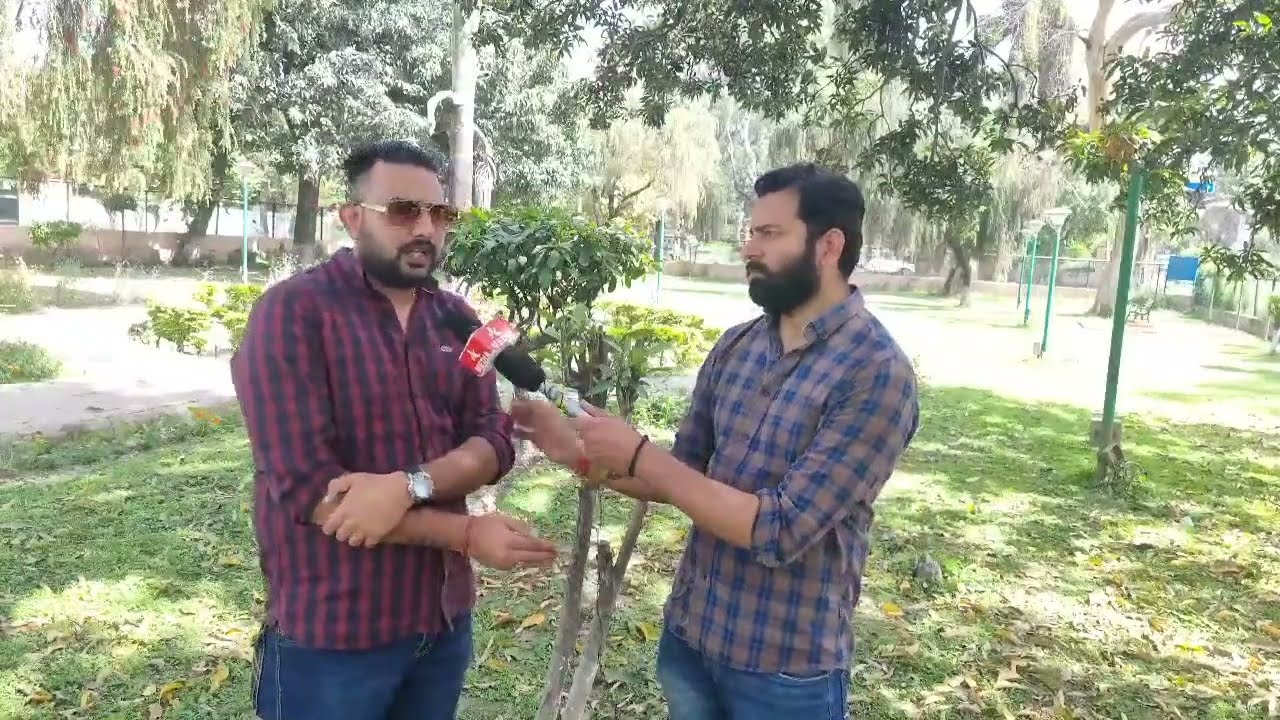In the photograph, two men are engaged in an outdoor interview in a scenic park setting. The interviewer, positioned on the right, has short black hair and a full dark beard, and is attired in a blue and gray plaid button-up shirt with blue jeans. He also sports a bracelet on his left wrist. Holding a black microphone with a red handle out towards the interviewee, he attentively listens.

The interviewee, standing on the left, features slicked-back black hair, a black mustache, and a short beard, and he shades his eyes with sunglasses sporting a gold frame and a brownish tint. He is dressed in a red and black plaid shirt, blue jeans, and a wristwatch on his left wrist. His left hand is gripping his right forearm as he speaks, mid-sentence, into the extended microphone.

Surrounding them, the park has a lush green grassy field dotted with various trees, many with vibrant green leaves despite their modest height of around 4 1/2 feet. Above and behind them, several green light poles with white tops line the scene. The background reveals more sparse greenery, faintly visible cars, and possibly a parking lot, all under an ample light-filled sky.